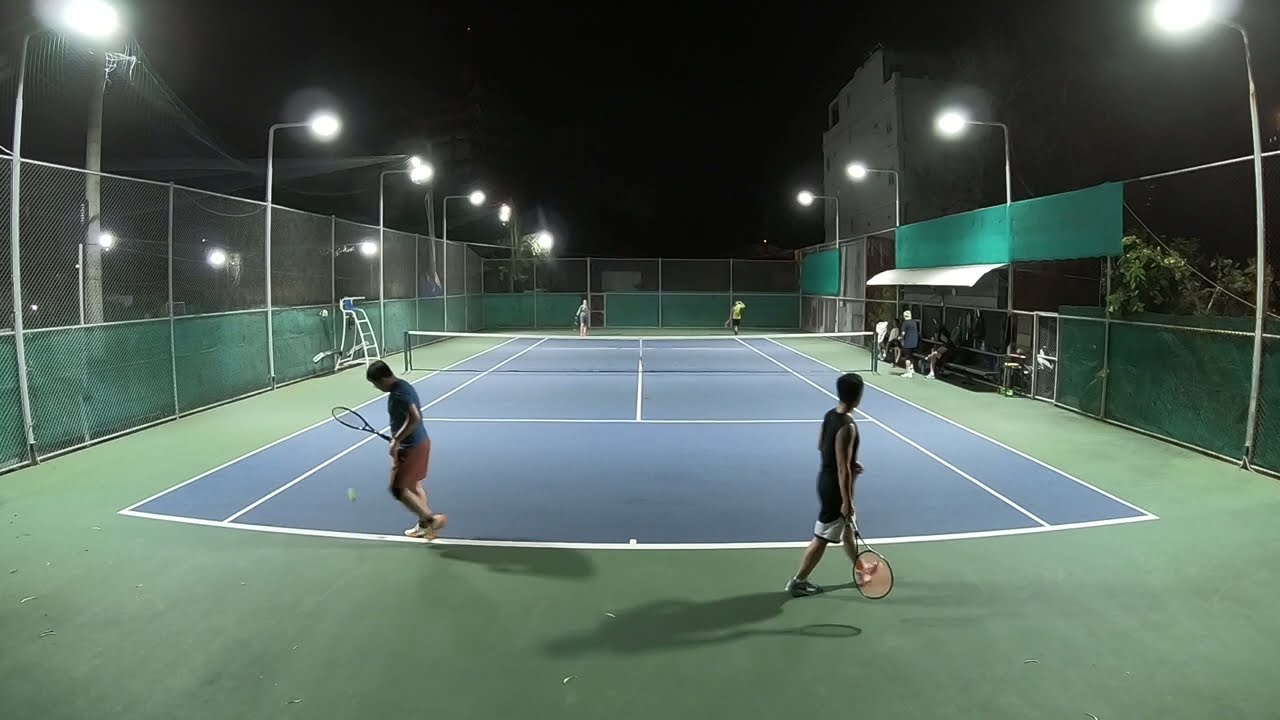This nighttime photograph captures an outdoor tennis court illuminated by tall lampposts with white lights that hang over the court. The court surface is blue with white lines and bordered by a green perimeter. Enclosed by green netting on the lower part and regular mesh fencing on the upper part, the setting hints at a possible college stadium, given a building in the background that resembles a college dormitory.

Four individuals are engaged in a tennis match, with two players on each side of the net. On the left side of the court, a man is bouncing a tennis ball, preparing to serve, while on the right, another man walks toward the end of the court. The players have distinct attire: one has an orange tennis racket with a black shirt and white shorts, while another carries a black tennis racket and wears a blue shirt with red shorts. The opponents at the far end of the court include one partially visible player in a yellow shirt.

Additional details include a ladder on the left side of the court, and on the right, there are benches under a small awning where a few spectators sit, watching the game. The court’s overall setting under a black night sky accentuates the lively activity happening on the brightly lit court.